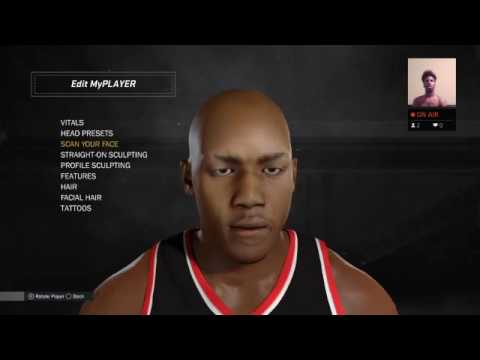This image is a screenshot from a video game featuring a character customization screen. At the center of the screen stands a basketball player, a black male with a shaved head, dressed in a black jersey with red trim along its borders and edges. Positioned at the top left corner of the screen is a button labeled "Edit My Player" in white text on a dark grey background. Beneath this button, various customization options are listed, including "Vitals," "Head Presets," "Scan Your Face," "Sculpt," "Straight On Sculpting," "Profile Sculpting," "Features," "Hair," "Facial Hair," and "Tattoos." Additionally, a smaller picture of another black male, seemingly shirtless, is visible in the upper left section of the screen.